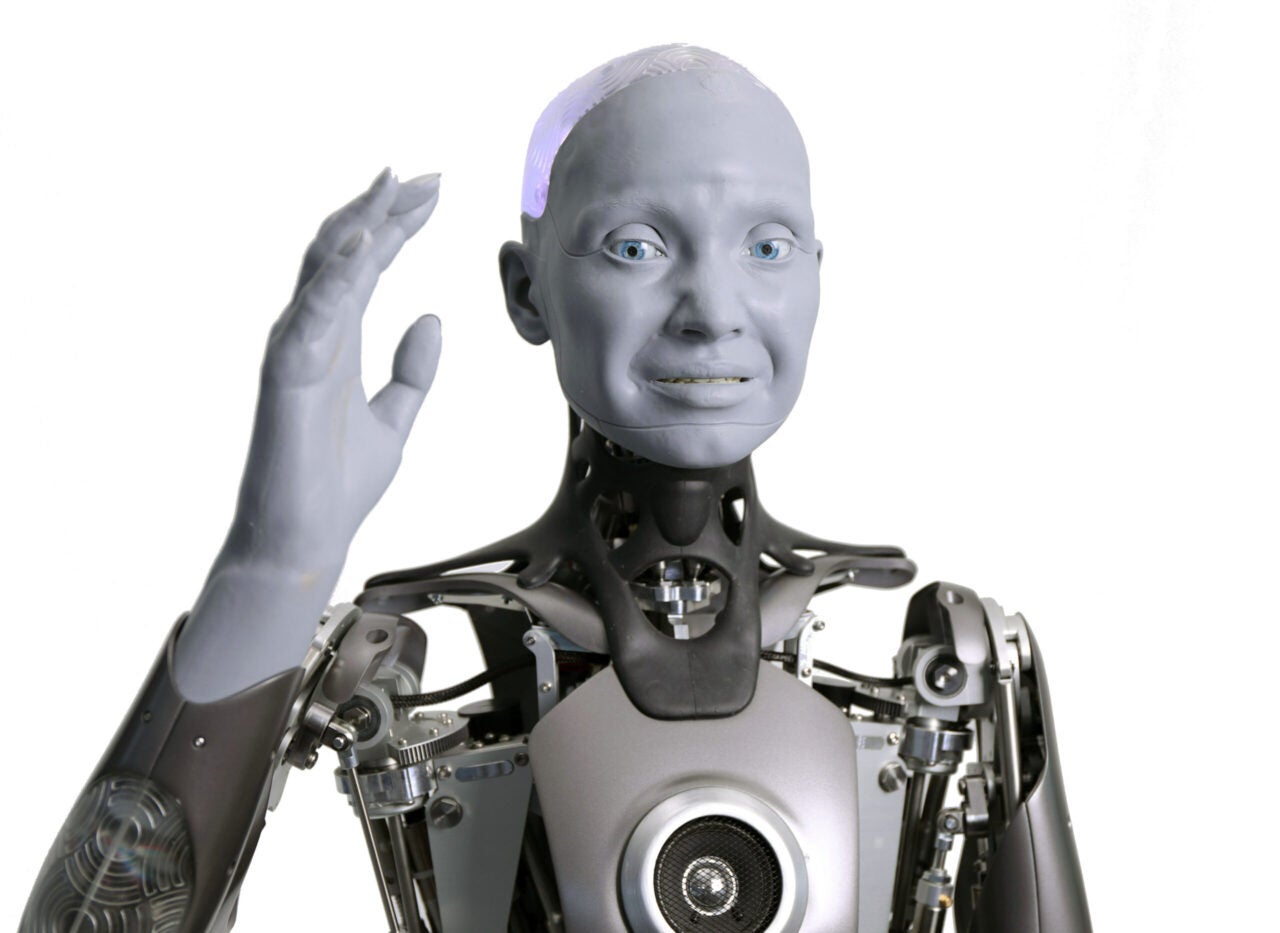The image portrays a modern, surreal depiction of a cybernetic robot with an anatomically human-like yet distinctly artificial appearance. The robot, highlighted from its chest upwards, features a sleek chrome and black silicone frame that cohesively connects its various parts. Its head, primarily illuminated in pink, presents a lifelike grey face with expressive, piercing blue eyes that gaze directly at the viewer. The head is bald and encased in a mix of black silicone and metal, adding to its futuristic aesthetic. Its right arm is raised, with the transformation from a blue-colored hand up to the wrist into a complex assembly of chrome metal and gears. The chest area features a prominent chrome plate with a central speaker, flanked by intricately visible gears and pistons. The shoulders are transparent, providing a glimpse into the robot’s intricate inner workings.